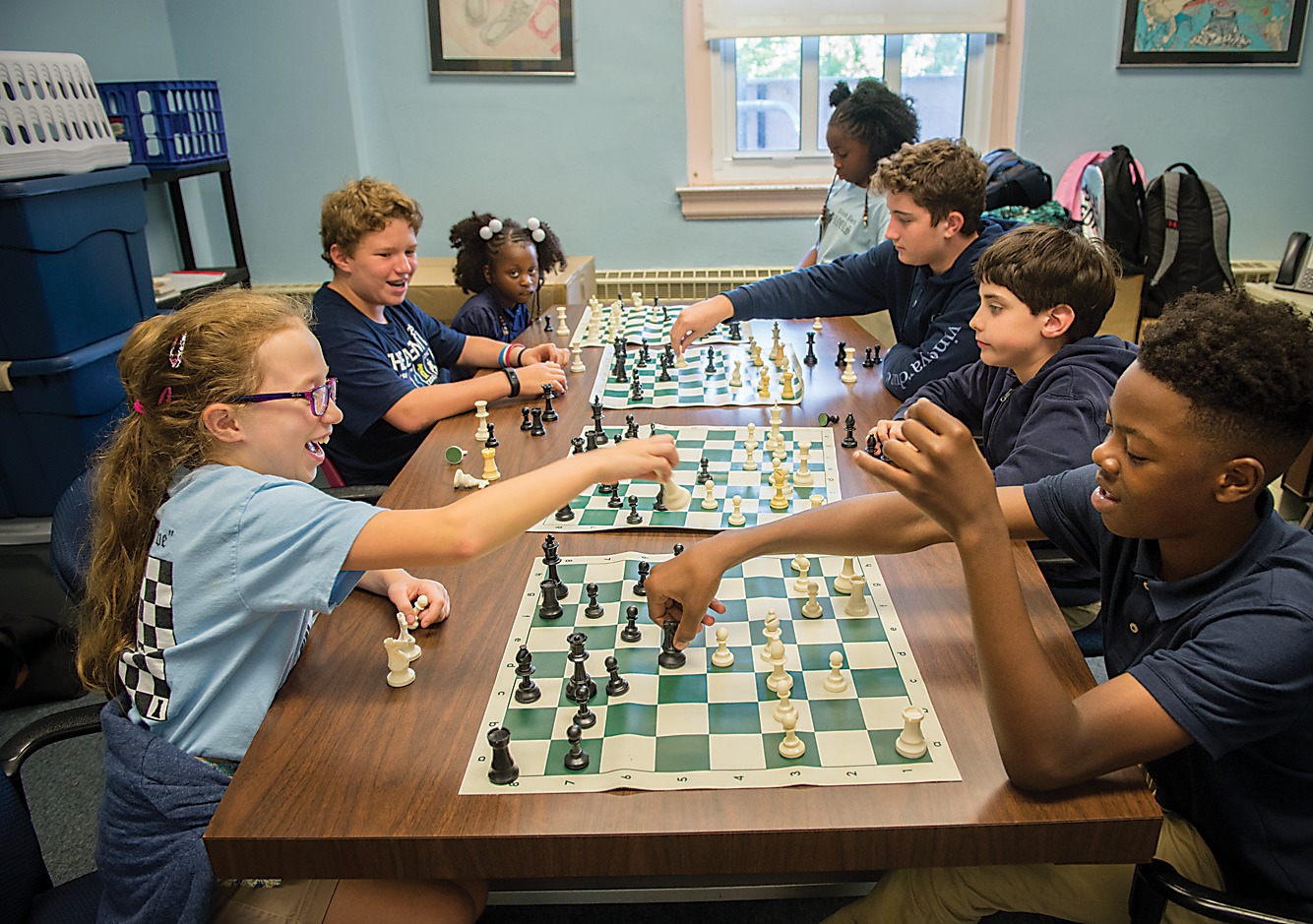In a bustling classroom setting, seven kids are engaging in a lively chess club session. Seated across a long wooden table with four tan and green checkered roll-up chess mats, the students are immersed in their games. On the left side, three kids are playing, while the right side has four participants, including one spectator. Their ages appear to be around ten, and they are dressed in various shades of blue, from lighter tones to navy. A mix of black, pink, and green backpacks are scattered in the background, alongside blue storage boxes stacked behind the kids on the left. Amidst the focused gameplay, smiles and a sense of enjoyment are evident, with a girl donning a t-shirt featuring a chess board, highlighting the group’s shared enthusiasm for the game.